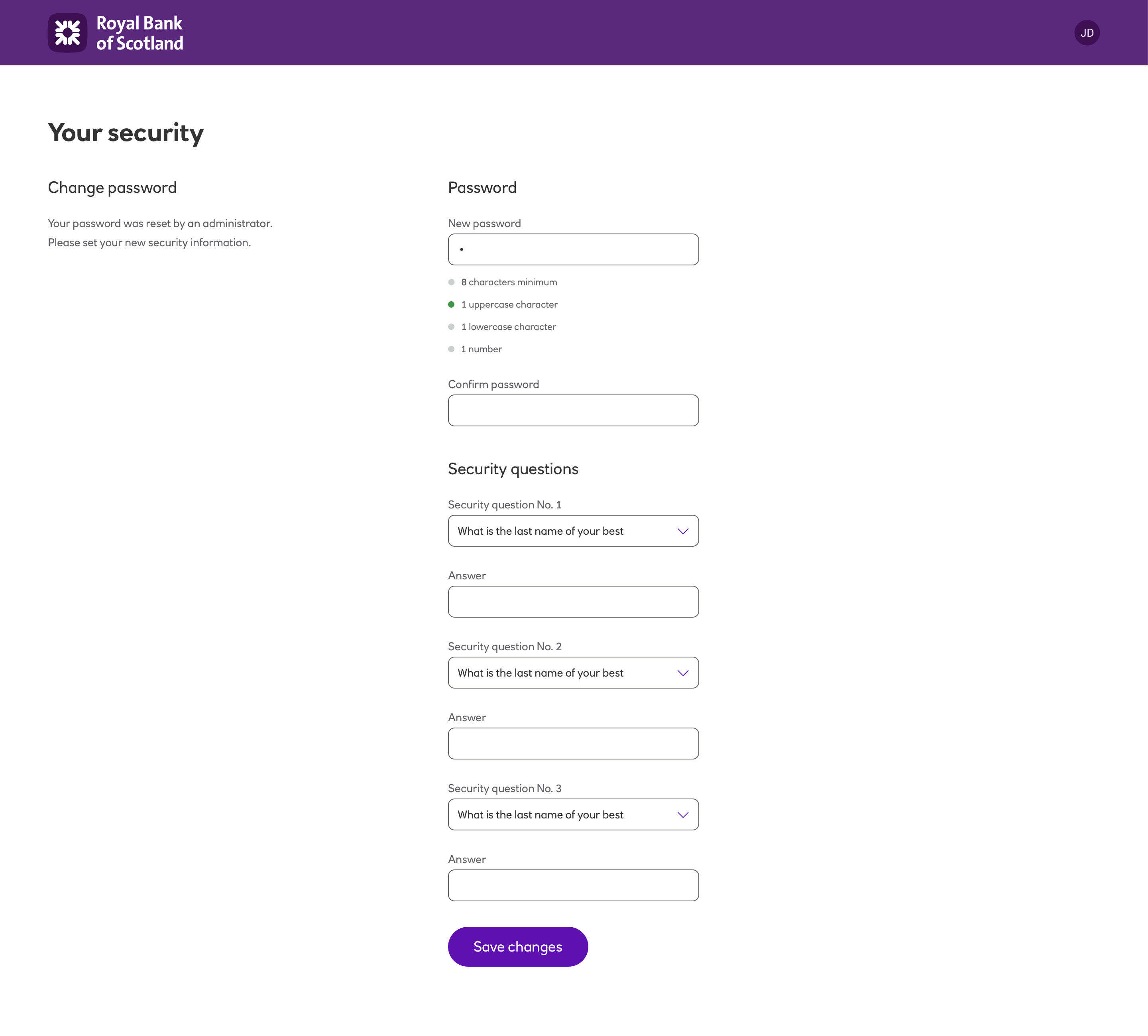Screenshot of a Royal Bank of Scotland Website Password Reset Page:

The image depicts a screenshot from a Royal Bank of Scotland website, featuring a predominantly solid white background. Dominating the top of the page is a not-very-tall banner in a deep royal purple color. Situated on the left side of the banner is the bank’s logo, which consists of a square formed by four inward-pointing white arrows set against a darker purple background. To the right of this logo, in crisp white text, is the name "Royal Bank of Scotland."

In the top right corner, there is a small, dark-purple circle containing the white capital initials "JD," indicating that a user with those initials is currently logged in.

The layout of the webpage is divided into three columns. The right column is entirely blank. The left column contains a main header in bold black text reading "Your Security," followed by a subheader "Change Password" in a slightly smaller font. Beneath this subheader, in an even smaller font, is a notification stating, "Your Password was reset by an administrator. Please set your new security information."

The center column is dedicated to the password reset form. At the top, there is a header labeled "Password," followed by fields to input and confirm the new password. Below this section is another header stating "Security Questions," accompanied by spaces to provide answers to three security questions. The placeholder questions displayed are all "What is the last name of your best?" which appears to be a placeholder error. There are drop-down menus available to select different security questions.

At the very bottom of this section, there is a purple button labeled "Save Changes," inviting the user to finalize their updates.